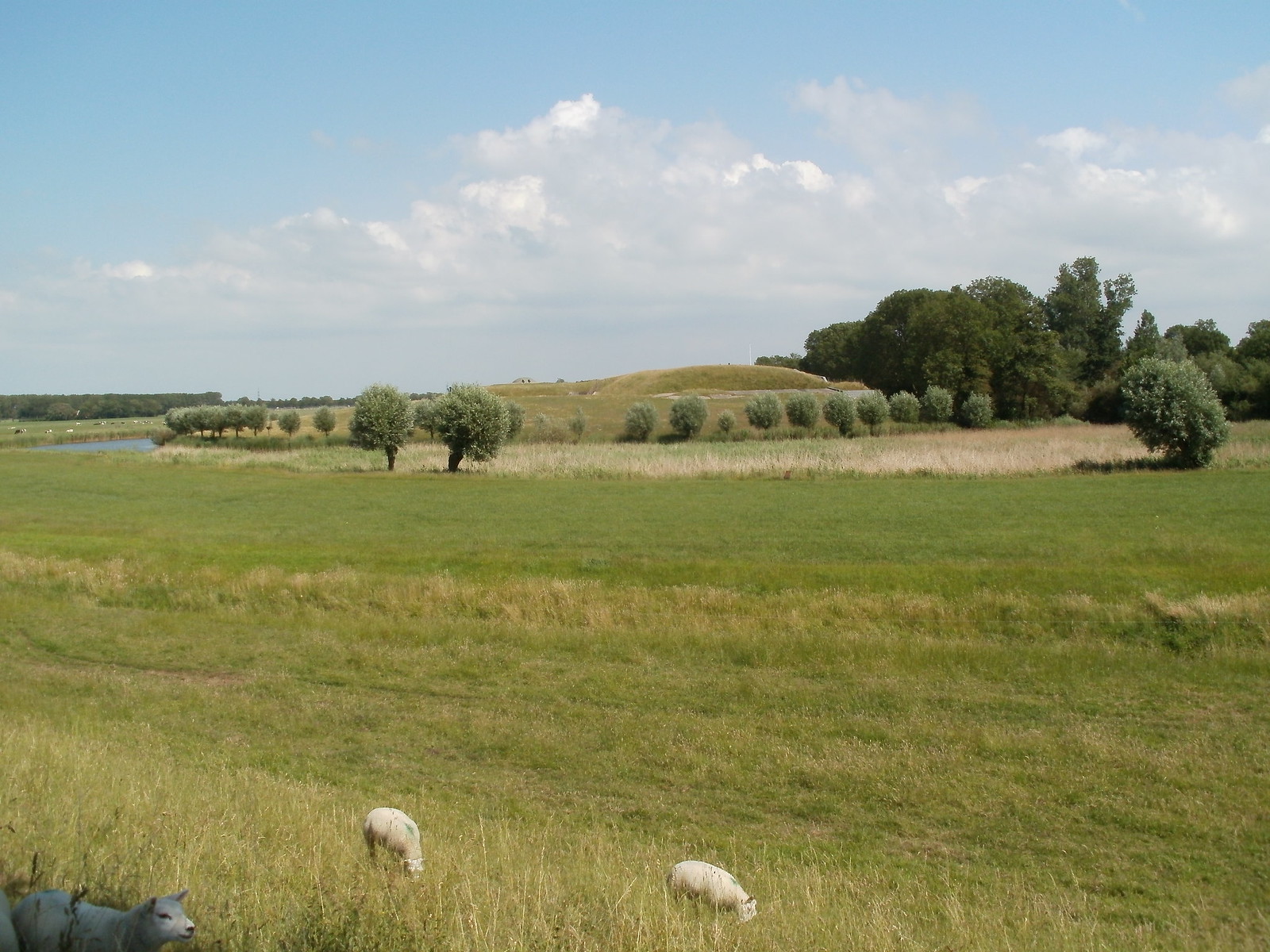This photograph showcases a serene countryside landscape featuring a vast, predominantly green grassy area with varying hues—from bright and light to dark green. Interspersed throughout the field are several lambs, two white and one gray, grazing contentedly on the grass. An additional lamb can be seen in the bottom left corner. The backdrop is adorned with a diverse array of trees and bushes, including short, small, tall, large, and thick trees in both light and dark green shades. A small rolling hill is visible in the distance, contributing to the picturesque scenery. Enhancing the tranquility of the scene, a tiny body of water is barely discernible to the left. Above, the sky is a vivid blue, dotted with numerous thick, white clouds, completing the idyllic rural vista.